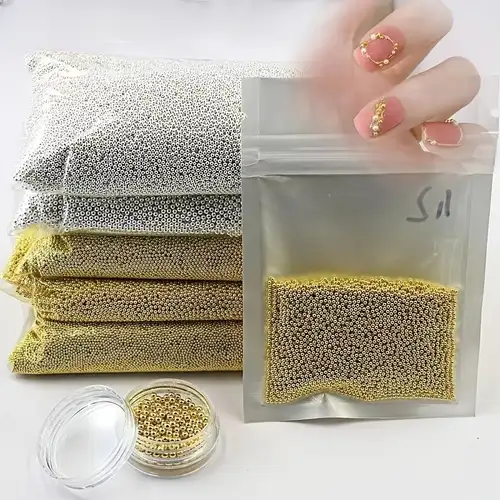The detailed, vertically rectangular, full-color photograph appears to be taken indoors under artificial lighting, with a plain gray background. It features a close-up display of small metallic beads, often referred to as BBs. In the upper right corner of the image, a woman's hand with thin fingers extends into the frame. Her fingernails are painted a shade of light pink, each adorned with delicate gold designs, echoing the beads' color.

The hand is holding a clear plastic bag filled with gold-colored BBs, which also has black text reading "SA." Additionally, scattered across the middle right section of the image are three more bags of gold BBs and two stacked on top of those, containing silver BBs. 

In the lower left corner, we see a small, circular glass jar filled with these same gold BBs with its lid removed and resting beside it. The arrangement of the products, combined with the carefully manicured hand, suggests a staged setting intended to showcase the BBs' potential use, possibly for decorative purposes such as nail art. The overall colors present in the image include shades of gold, silver, gray, beige, pink, and white.